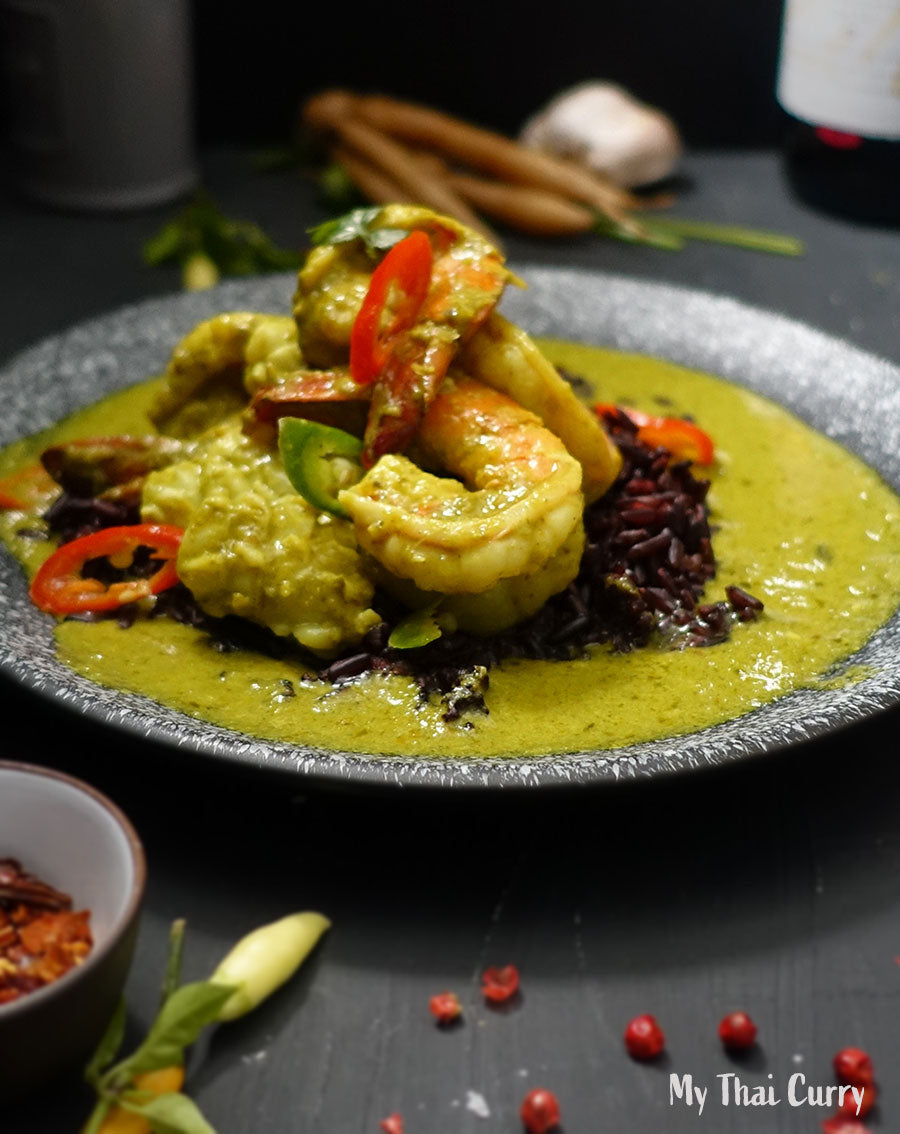A close-up photograph captures a mouthwatering Thai curry dish served in a stylish, gray and white speckled bowl. The vibrant yellow curry is richly adorned with succulent shrimp, red and green bell peppers, and whole peppers that add a burst of color and flavor to the composition. The lower-right corner credits "Mai Thai Curry" for this delectable creation. The foreground features additional bowls filled with whole peppers, enhancing the culinary theme. Out of focus in the background, various bottles and perhaps more peppers are subtly visible, adding depth and context to the dining setting. This visually appetizing scene beautifully showcases the artistic and flavorful essence of Thai cuisine.